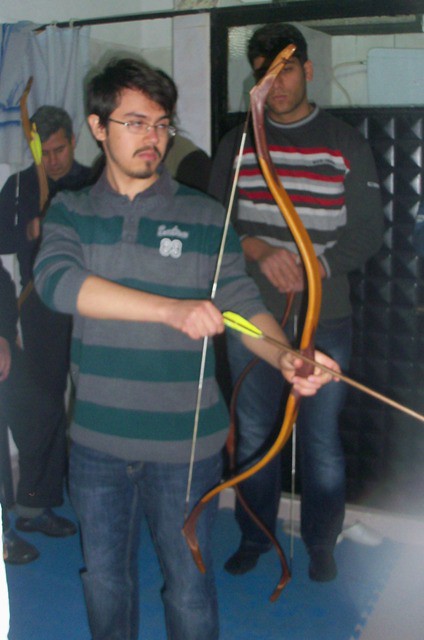In the image, a group of three men are standing in what appears to be an indoor archery range, characterized by a white wall and possibly black lockers in the background. The focus is on the man closest to the camera. He has black, short hair, glasses, a light beard, and a goatee. He is dressed in a gray and blue striped shirt with an indistinct white symbol on the top right of his shirt and blue jeans. He is holding a simple wooden bow, positioned to his right, with an arrow fitted but not fully drawn, and yellow fletching on the arrow.

Behind him stand three more men. The man directly behind and mostly obscured is holding his bow with an arrow, which has similar coloring to the one in front. To his left stands a shorter man dressed in all dark blue or black. This man is also holding a bow. On the far right, the tallest of the three men is visible, wearing a red and white striped shirt with gray sleeves and blue jeans, his bow resting on the ground. He stands with his hands together watching the man in front. 

All three men in the back seem to be observing or preparing to take their turns. The scene suggests they are all part of an archery activity indoors on a carpeted floor, with the front man in the middle of aiming his bow.